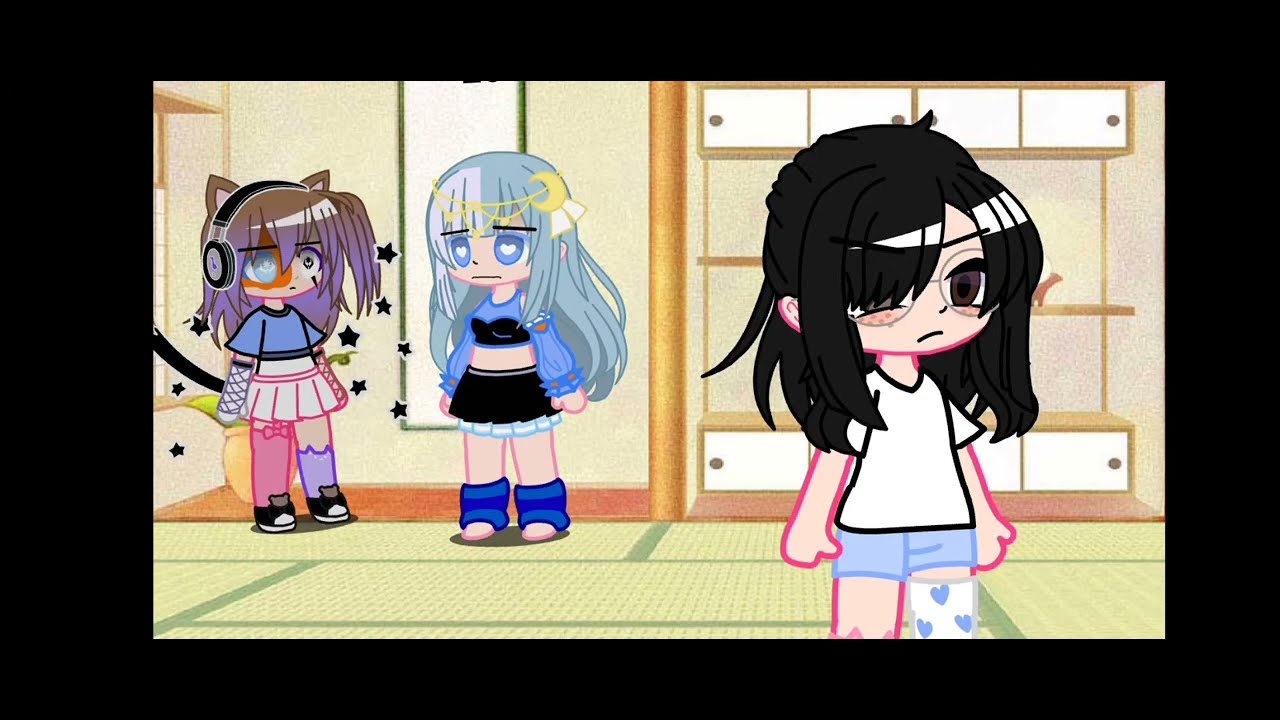The detailed color cartoon image has a thick black border, especially prominent on the sides. Depicted are three cartoon girls in a room with light yellow and gray tatami mat flooring outlined with green borders, giving an Asian aesthetic. The setting includes a white wall with cabinetry, possibly wooden, in the background, and a green-framed mirror against the beige or light green left wall.

The girl on the far right, closest to the viewer, stands out with her long black hair, parted to cover one eye partially, and thin-rimmed glasses on her face. She wears a white shirt, short blue shorts, and a white cast decorated with blue hearts on one leg. She faces slightly to her right, showing only one purple iris clearly.

Behind her, to the left, are two girls standing close to each other. The middle girl has long blue hair with bangs, eyes shaped like blue hearts, and a solemn expression. Her attire includes a black bustier top with long blue sleeves, a black skirt with white ruffle, and loose ankle warmers. She also wears a golden headpiece with a half-moon ornament.

The leftmost girl sports long hair that transitions from brown to purple, topped with cat-like ears. She wears a pair of oversized headphones, a blue short-sleeve crop top, a white skirt, and mismatched socks—one pink, one purple, complemented by blue shoes. Her outfit and expression suggest a sense of confusion.